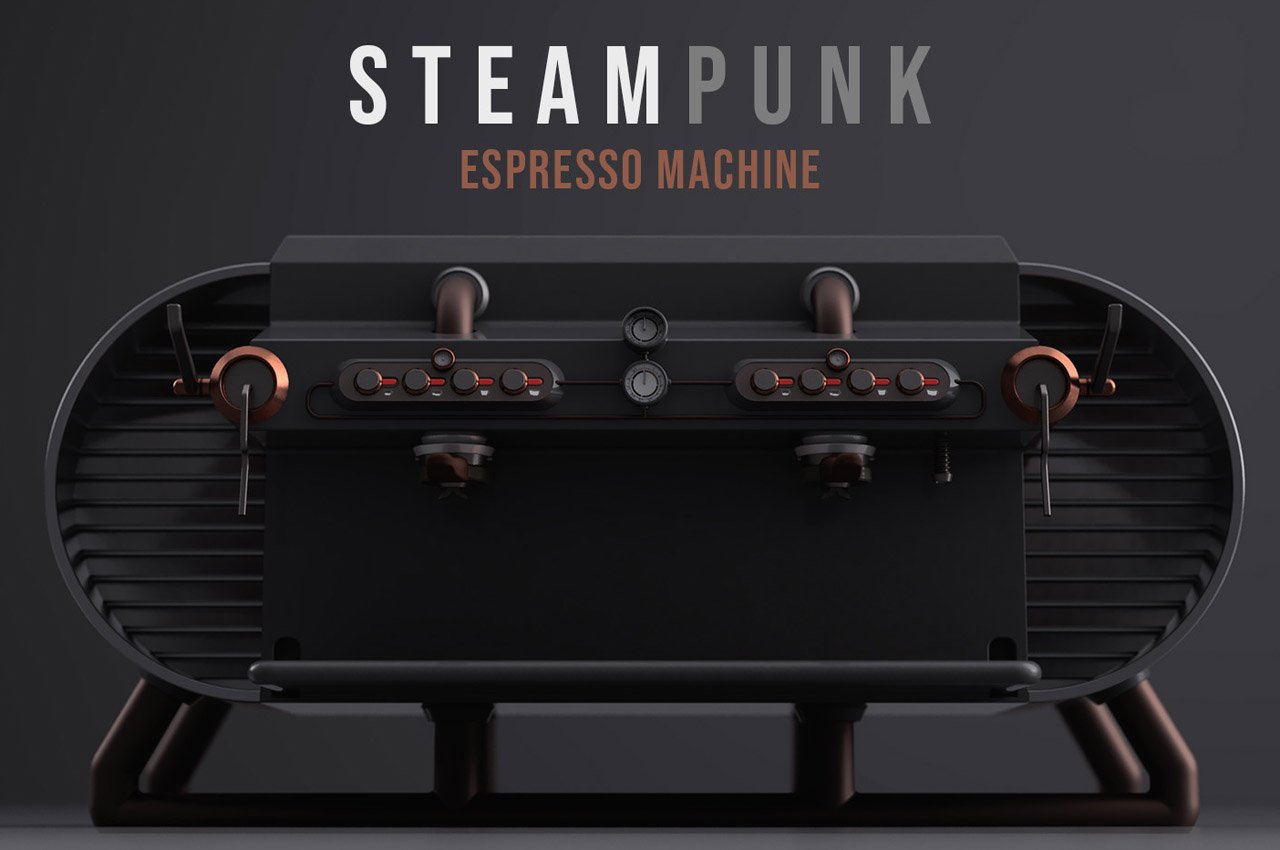The image features a visually striking, steampunk-themed espresso machine set against a uniform dark gray background. At the top, the word "STEAMPUNK" is prominently displayed in all capital letters, with "STEAM" in white and "PUNK" in a bluish-gray color. Directly below, also centered and in all caps, the words "ESPRESSO MACHINE" are presented in a brown hue. The espresso machine itself is capsule-shaped and appears meticulously designed, resembling an old-fashioned radio. It is symmetrically divided into two halves, enabling the simultaneous brewing of two cups of espresso.

The machine’s exterior is characterized by a gray body with ridges in the center and a series of intricate features. There are eight control knobs—four on each side—allowing users to customize their brewing preferences. Additional design details include a pair of brown tubes emerging from the top and a brass knob located at each end of the machine. At the bottom, there's a downward-facing spout and a small level platform where the espresso cups can be placed, supported by a dark brown, copper-like metallic base. This espresso machine embodies a steampunk aesthetic with its detailed and symmetrical design, enhanced by the sophisticated blend of colors and textures.